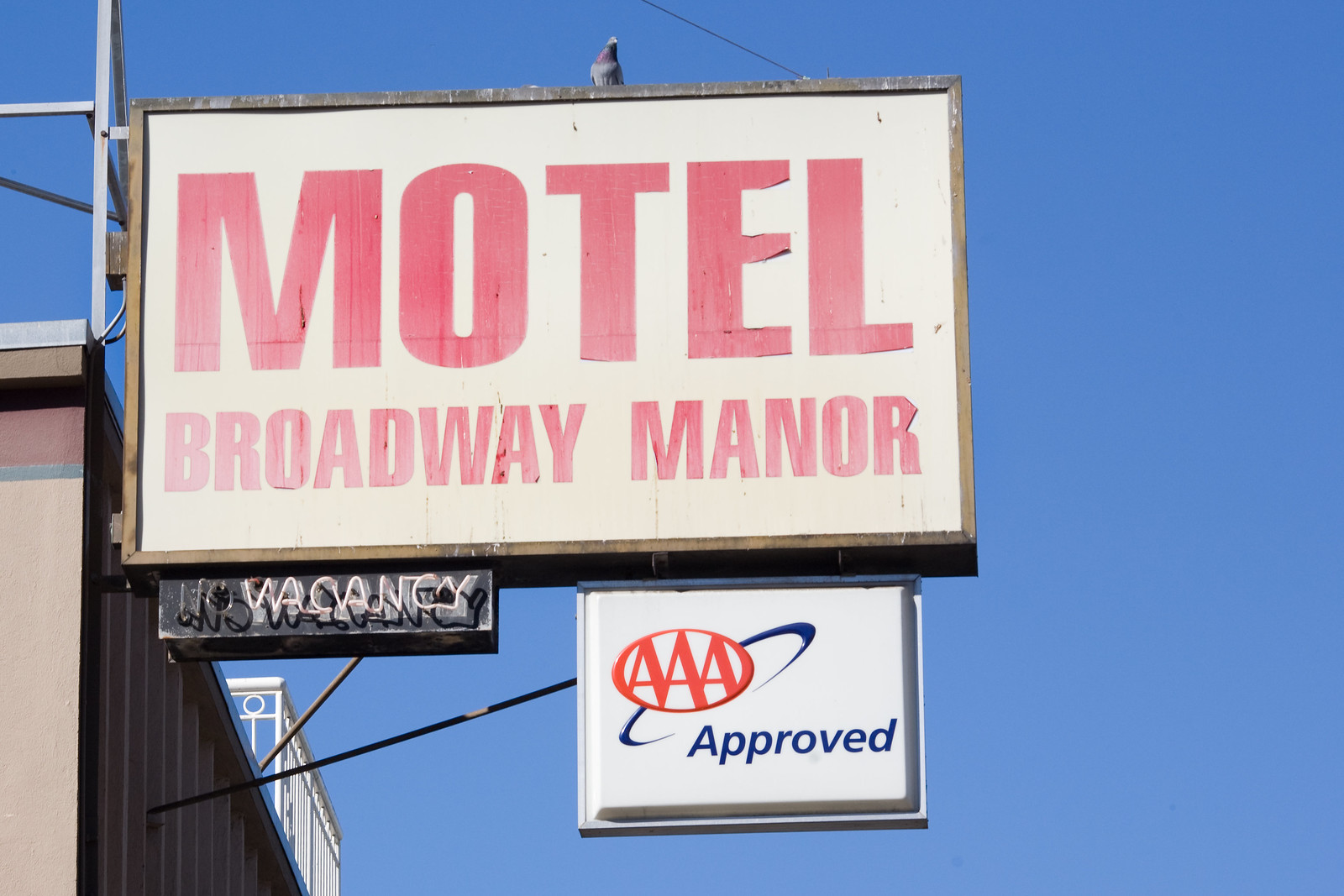The photograph captures a vintage motel sign situated on the side of a building against a crisp, clear blue sky. The sign, which has a white background with a slightly yellowed, worn appearance, features large, faded red letters reading "Motel Broadway Manor." The weathered text shows signs of age, with the "E" in "Motel" and the "R" in "Manor" notably peeling. The sign has a dark steel border and sits perched atop a dark beige and red-trimmed building, partially visible on the left side of the image. 

A brown pigeon is seen resting atop the sign, adding a touch of life to the scene. 

Hanging below the main sign are two additional signs: a white rectangular one displaying a red and blue "AAA Approved" logo, and a small black rectangle indicating "No Vacancy." The "No" in "No Vacancy" is unlit, while "Vacancy" glows brightly in white neon, suggestive of classic motel signage.

Visible below the signs are supporting poles and beams, alongside a white railing that forms part of the motel structure. The overall atmosphere is marked by the old-world charm of the weathered sign against the backdrop of a pristine, cloudless daytime sky.